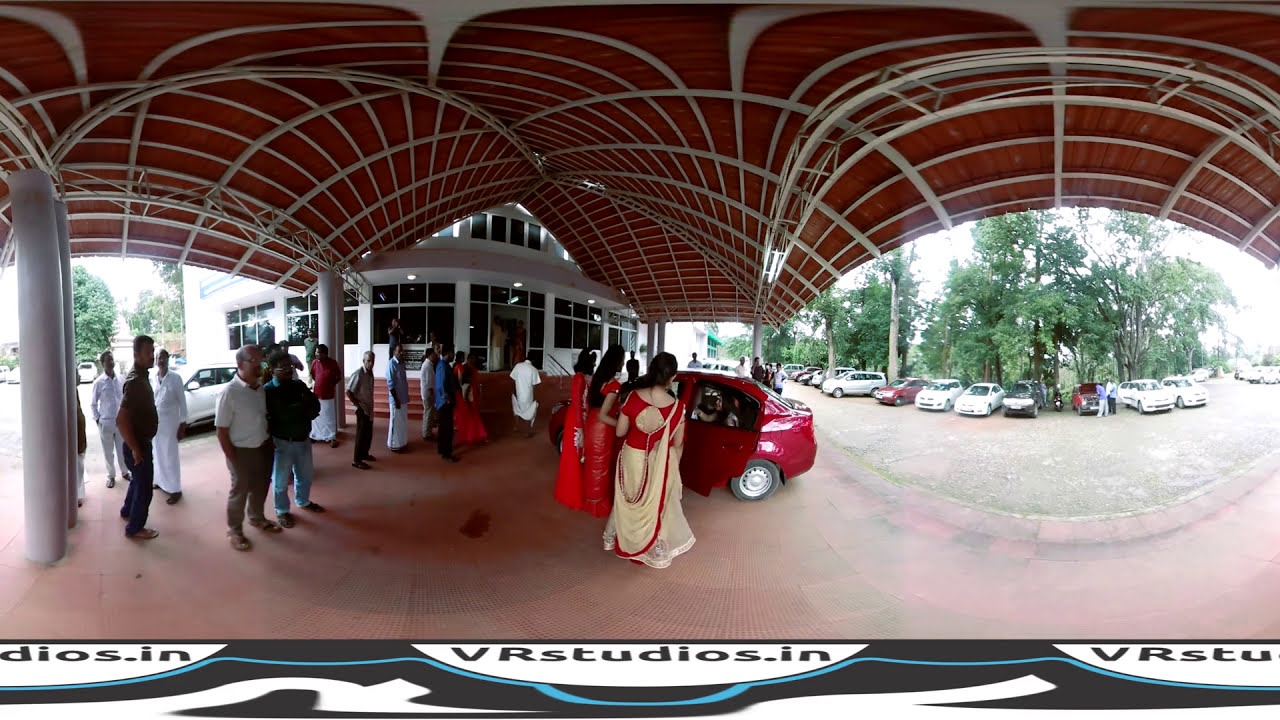The image is a panoramic photo of a scene set in front of a white building with glass windows and a distinctive red metal roof supported by a white framework. The building features awnings and an overarching curved roof design. In the center of the image, three women dressed in traditional Indian attire are gathered around a red car, engaging with a woman seated in the car's backseat through the open door on the left side. The lady in the backseat is being welcomed by the women outside. To the left of this group, several men are standing and observing the scene. Additionally, in the right section of the image, a few men are meticulously inspecting the engine of a vehicle in a parking space. The parking area around them is filled with cars, and behind the parking lot, a lush row of trees is visible. The ground in the area where the red car is parked has a reddish hue. At the very bottom of the image, there is a logo for VRstudios.in.